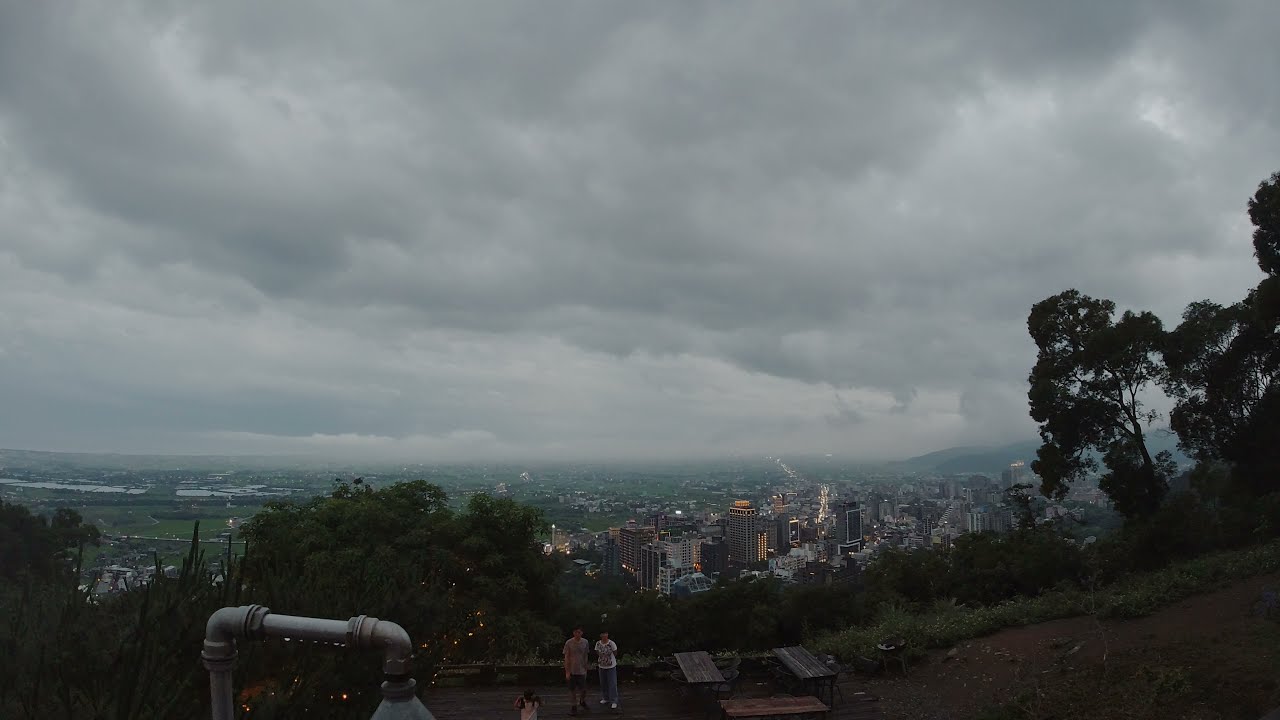This color photograph captures a rainy, overcast day from an elevated vantage point, likely taken from a hill or park overlooking a sprawling urban city. In the foreground, set against the backdrop of an expansive cityscape with numerous tall buildings and main roads, stand three people, two of whom are posing for the picture. They are positioned near two wooden picnic tables and a distinctive metal pipe shaped like an upside-down 'U'. The surrounding area features lush greenery with trees and patches of dirt indicative of the hillside terrain. Despite the dreary weather marked by dark gray clouds and perhaps some fog, the image provides a detailed view of the urban environment extending into the distance.